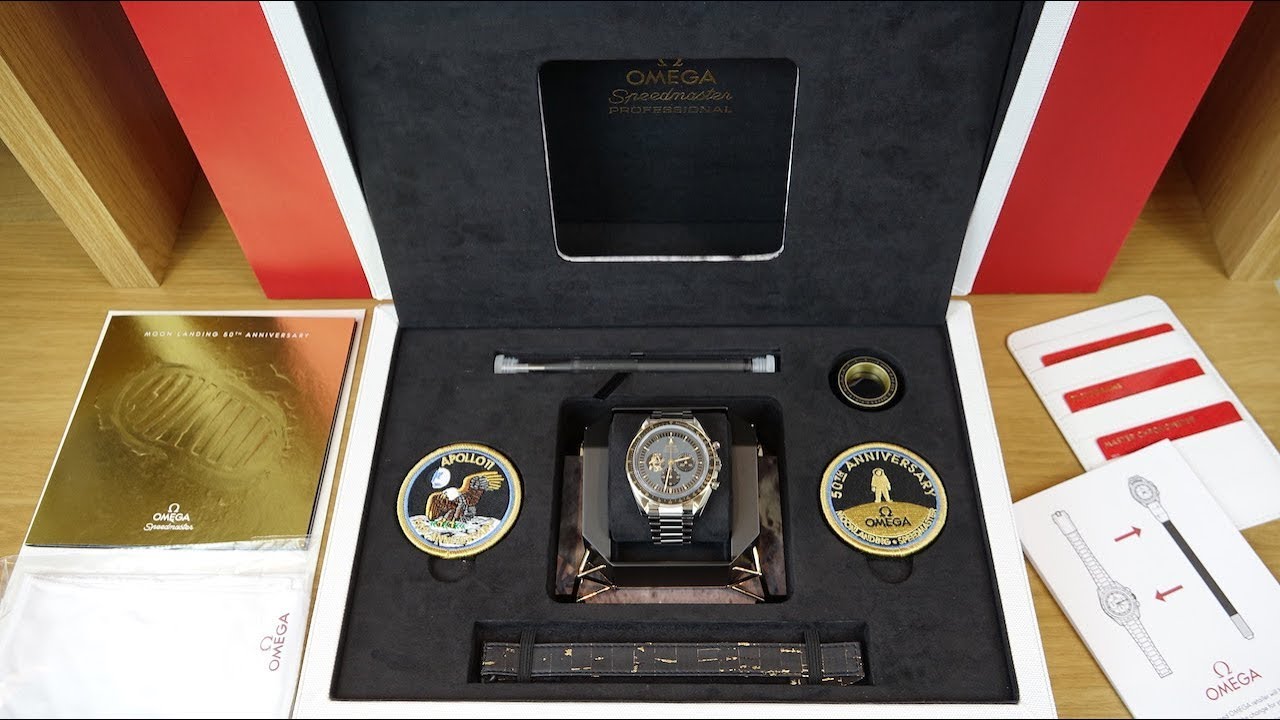This is an image of a highly detailed and elaborate boxed watch set by Omega, commemorating the 50th anniversary of the Apollo 11 mission. The watch set is encased in a luxurious presentational box with an Omega logo prominently displayed on the inside flap. The box features a sophisticated design with black velvet interiors and red trim. At the center of the box is a distinguished gold Omega watch, set meticulously on a velvet background within its own compartment. This watch is affixed with a metallic band, showcasing a blend of silver and darker gray metals typical of men's watch designs, although it could be unisex.

Flanking the watch on both sides are commemorative medallions. The medallion on the left honors the Apollo 11 mission, depicting an eagle landing on the moon's surface with Earth in the backdrop, encapsulated in a black background. The medallion on the right appears to signify the mission's 50th anniversary, illustrating an astronaut on the lunar surface with the Omega logo below. In addition to the watch and medallions, there is a long tool with white caps at either end set into the velvet case, possibly for adjusting the watch or its components. 

Below the watch is a strip that appears to be an alternate black leather watch band adorned with stellar markings, evoking constellations or celestial navigation charts. Alongside the box on the left is a gold-embossed pamphlet and to the right are several cards, presumably the owner's manual and instructional booklets detailing the watch's features and functionalities.

Overall, this Omega watch set melds elegance and historical homage, emphasized by its meticulous presentation and the accompanying artifacts celebrating one of humanity's monumental achievements in space exploration.